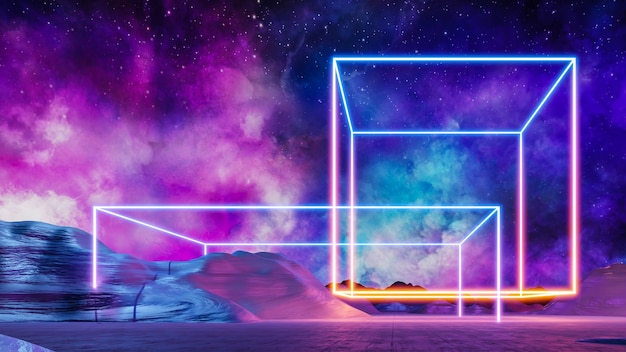This digital 3D rendering is a striking sci-fi skyscape featuring two neon-outlined squares of different sizes. The smaller square, prominent and closest to the viewer, has a dynamic gradient perimeter: its bottom starts in orange and morphs into an orange-purple vertical line, which then angles left to become a blue laser-like top line, finally descending into another purple segment. The larger square, glowing entirely in white neon, hovers over a smooth, reflective hill or sand dune-like structure. The ground gives off a reflective, smooth appearance, extending a flat surface interspersed with a somewhat reflective rocky formation on the left side.

The sky is a captivating moonlit scene with stars glistening against a black backdrop, framed by ethereal lavender clouds on the left and blue clouds on the right, with hints of pink hues intertwining throughout. This cool neon virtual reality space art seamlessly blends futuristic aesthetics with ambient celestial elements, creating a captivating and immersive visual experience.